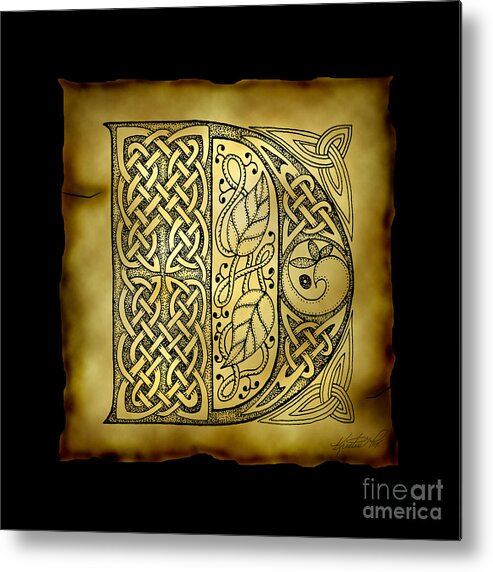This digital image showcases a highly detailed and intricate representation of the letter "D," adorned with traditional Celtic-inspired patterns featuring interwoven ribbon designs. The interior of the "D" includes intertwining stems and leaves, while the outer part continues the Celtic motif. The design appears to be a digital recreation, made to resemble a painted initial from old-style books of the 1500s. The letter "D" is set against a 3D-generated mock-up of aged manuscript paper, which lies on a black background, enhancing the historical feel. Additionally, the image bears the watermark "Fine Art America" in the bottom right corner, with varying font sizes and boldness, lending a subtle yet present branding touch.